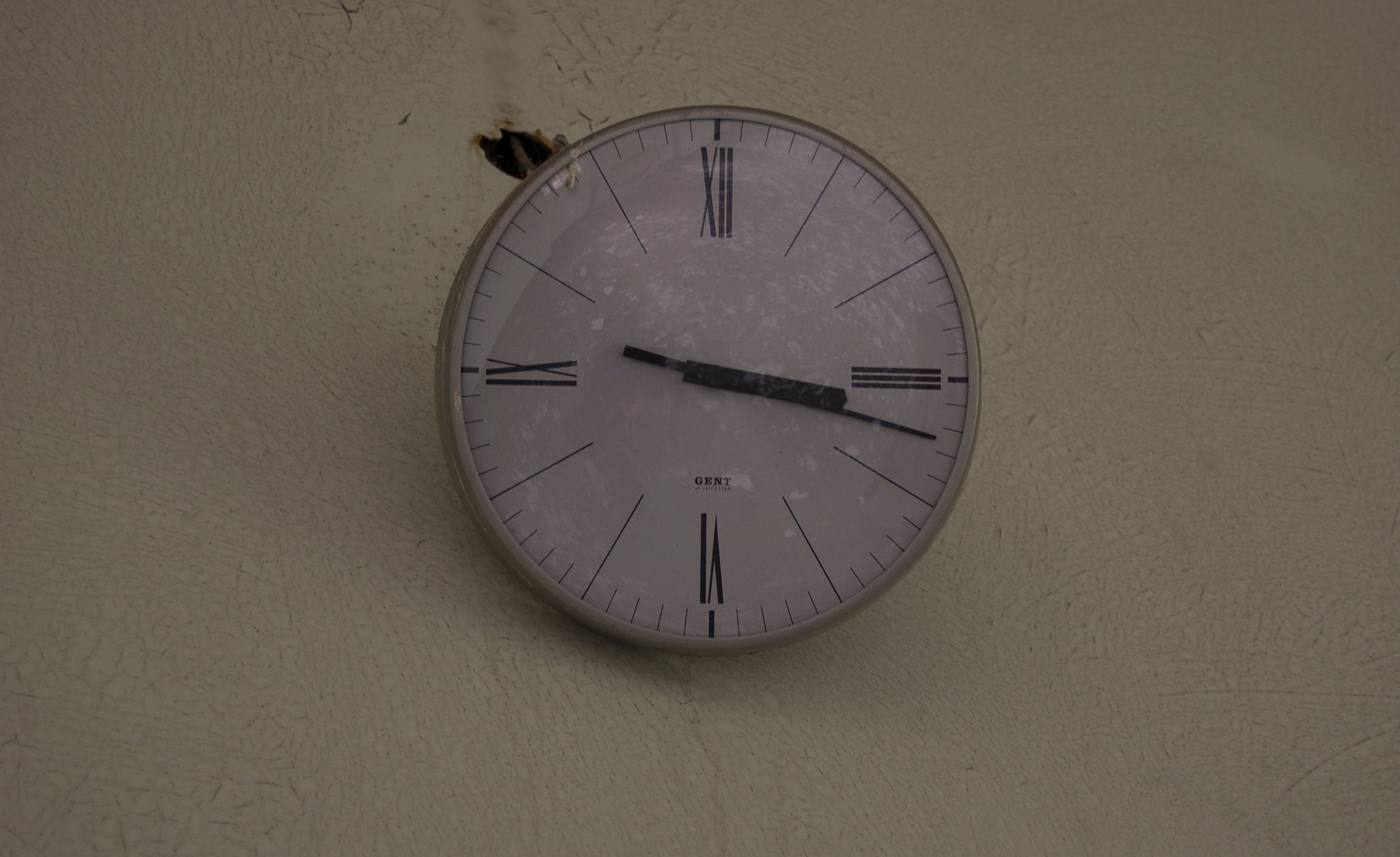The image features a clock prominently centered, set against a distressed off-white beige wall riddled with cracks, indentations, and spots, indicative of an aged or worn surface. The clock face is white, encircled by a silver rim. Notably, it displays Roman numerals only at the 12, 3, 6, and 9 positions, specifically 'XII', 'III', 'VI', and 'IX'. The remaining hours are marked by slender black lines, while traditional short black lines denote the minutes. The clock's hands are also black. At the center of the clock face, there's the word "GENT" printed. Peering closely, a background detail reveals a hole or burnt spot behind the clock, with some exposed wires, suggesting it might be slightly detached from the wall. There is also a faint reflection on the clock's glass surface, hinting at possible outdoor elements like trees, though it remains ambiguous.